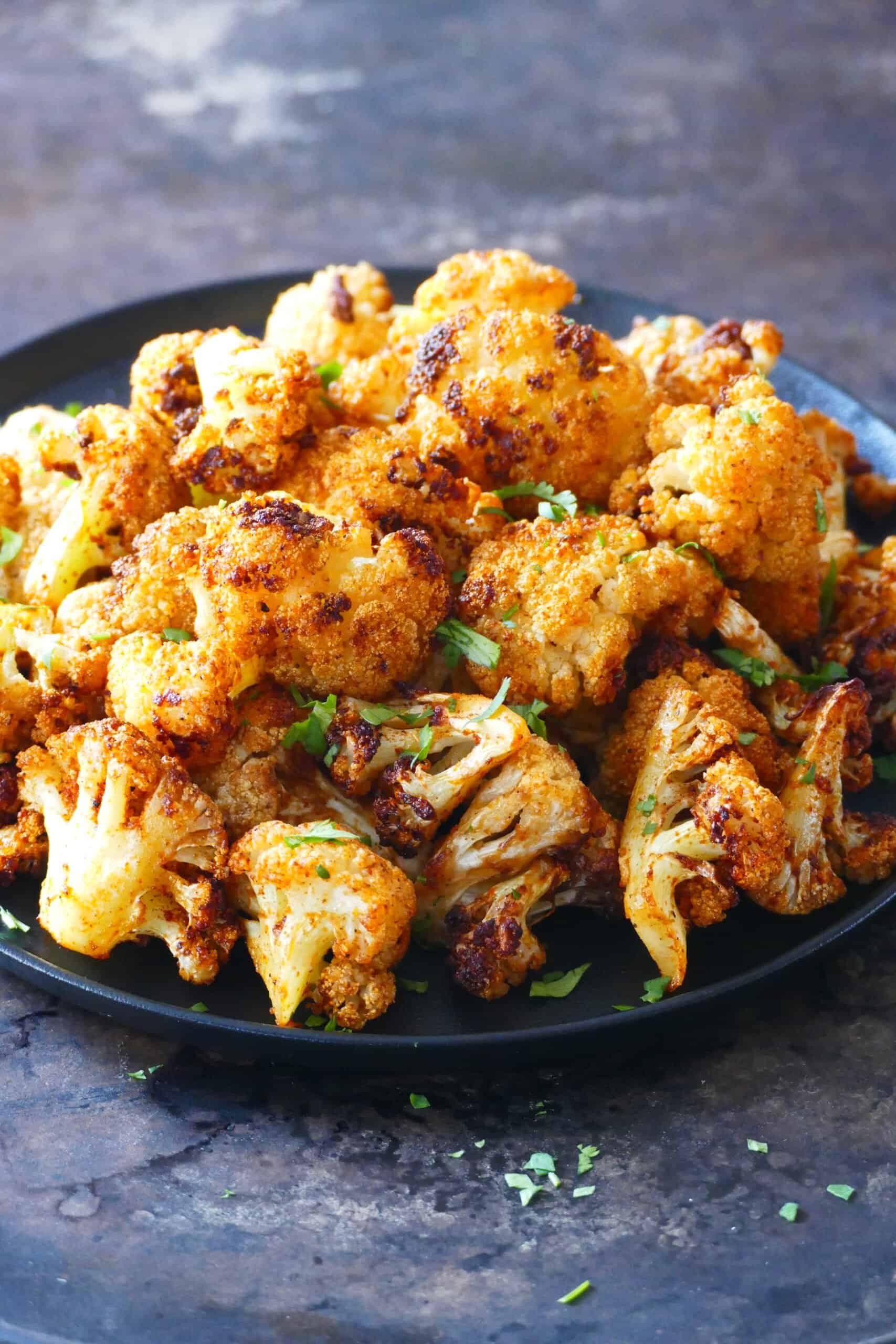This is a photo-realistic, vertical close-up image of a black plate filled with approximately 19 pieces of grilled cauliflower, artistically arranged and garnished with shredded parsley. The cauliflower, which might be intended as a buffalo-style dish, has a range of coloring from golden to deeply browned with some edges appearing almost charred, hinting at its crispy texture. The black plate is placed on a brown or black marble countertop, with some pieces of parsley scattered carelessly on the plate and the marble surface. The shot is taken from a 45-degree angle, focusing on the plate, leaving the background out of focus, and emphasizing the rich details and textures of the grilled cauliflower.